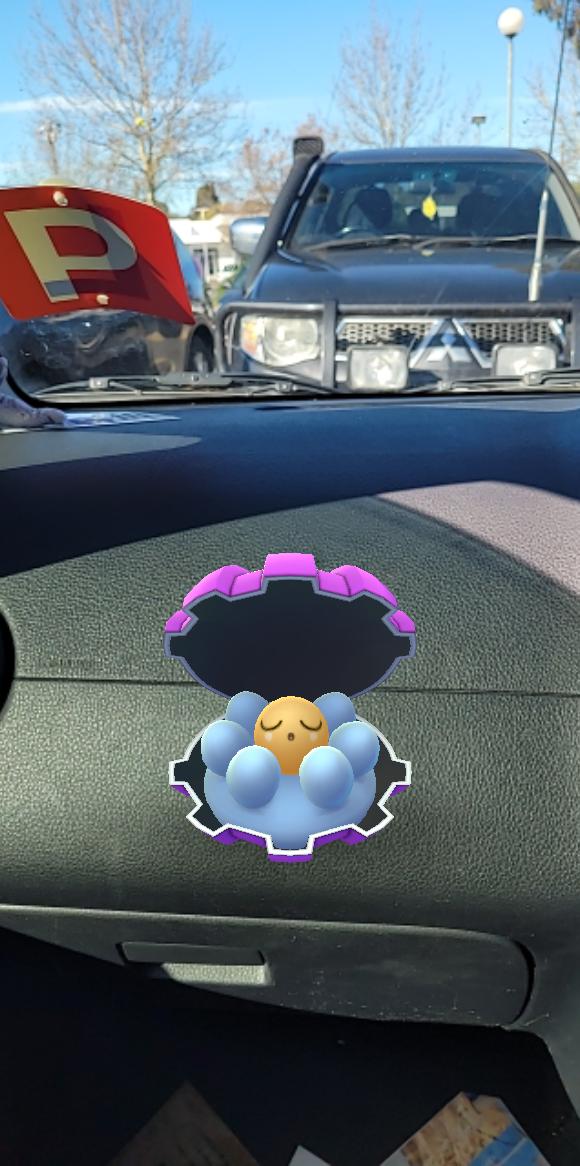This detailed image captures the interior and exterior views from the passenger side of a vehicle. The focal point inside the car is a dark gray dashboard with an AI-generated image resting on it. This image is clamshell-shaped with squared-off ridges around the edge. It features a central round blue object surrounded by white balls on the outer edge, and a bigger central yellow ball with two downward-facing C-shaped eyes, resembling a sleepy or abstract face. The glove compartment and its black handle are visible beneath the dashboard, revealing some clutter on the floor with yellow and blue wrappers.

Peering through the windshield, there are various external details. A prominent red square sticker with a bold, uppercase white 'P' is affixed to the windshield's upper left corner. Through the clear windshield, a black truck is seen facing the vehicle, identifiable by its black and silver Mitsubishi logo, a distinctive triangular shape, and a yellow air freshener hanging from its mirror. The truck's headlights are partially visible, with one large and two smaller ones apparent. Surrounding the scene, a vivid blue sky and several bare trees with brown trunks and branches set the background, highlighting the contrasting colors in this comprehensive and intricate snapshot.